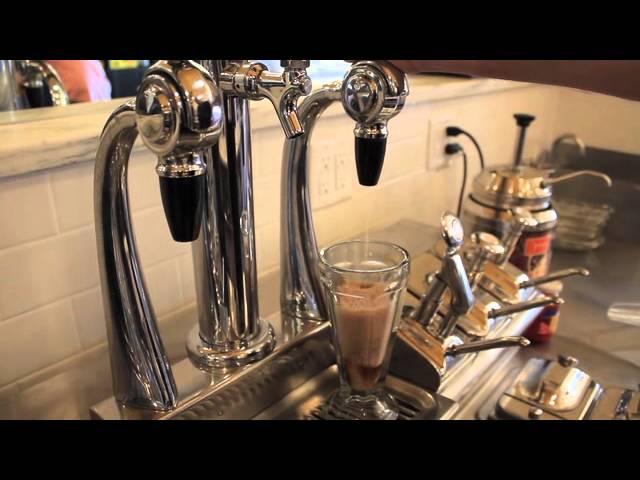The image is of a modern soda fountain setup akin to those in an ice cream parlor. Central to the photograph are three chrome dispensing taps arranged in a line, two of which feature black nozzles for flavored soda, and a central tap that appears to dispense plain water. All taps emanate from cylindrical, silver-colored pipes anchored to a chrome base, which includes a drainage plate. Positioned on the drainage plate is a tall, tapered glass filled with a foamy dark brown liquid, likely a root beer float or a similarly styled beverage. To the left of the taps, on the viewer's right, there are syrup dispensers with taps for adding flavors to drinks or ice cream. Further along, towards the edge of the counter, there is a metallic tank with a long spout—possibly a hot fudge dispenser—topped with a plunger for dispensing the fudge. The backdrop is a white, cinder-block wall featuring several electrical outlets with plugs connected. Additional elements include ladles and metal containers potentially holding ice cream toppings, hinting at the soda fountain's role in crafting various desserts. The photograph is bordered by broad black bands at the top and bottom, adding to its polished presentation.